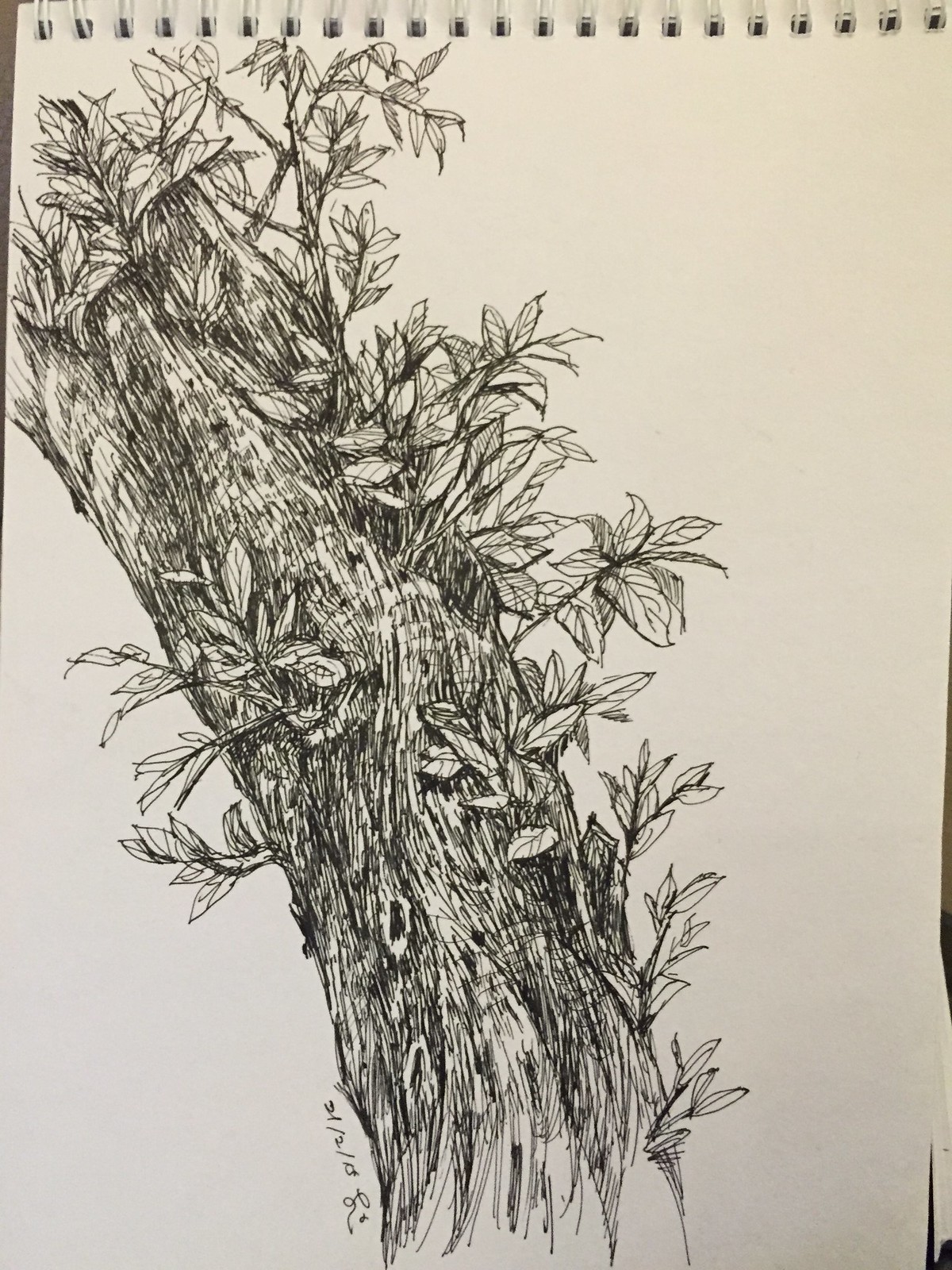The illustration depicts a detailed black ink drawing of a tree branch, complete with delicate leaves sprouting from the wood. The artwork is showcased on the pages of a flip journal, presenting it as an elegant sketch. In the lower-left corner of the image, a date is inscribed, adding a personalized touch to the piece.